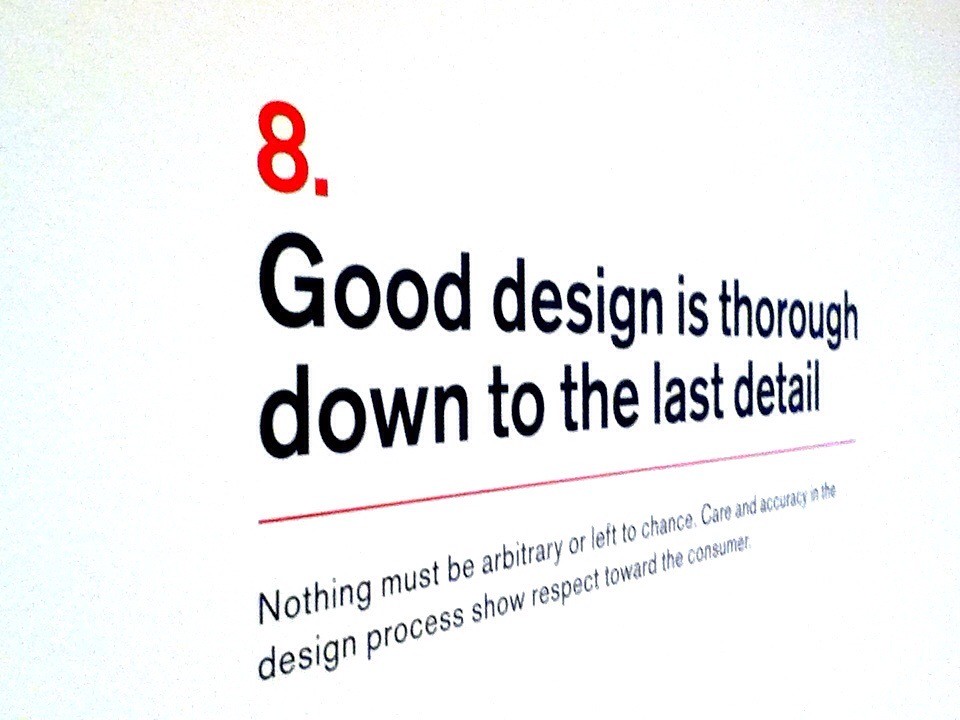The image features an entirely white background with a slight grainy gray texture along the sides. At the top of the image, a red number "8." followed by black text reads "Good design is thorough down to the last detail." The top section's text size gradually decreases from left to right and appears to be slanting downward. This text is separated from the lower section by a thin red line. Below the line, smaller black text that also decreases in size from left to right and slants upwards reads, "Nothing must be arbitrary or left to chance. Care and accuracy in the design process show respect toward the consumer." The overall layout gives a 3D effect, making the text appear as though it is receding into the distance. This conveys a sense of meticulousness and precision, highlighted by the consistent theme of careful design presented in the text.